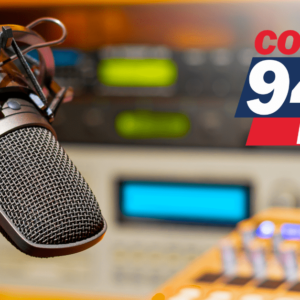The image captures a detailed scene inside a high-end music or recording studio, potentially part of a local radio station, with a professional-grade silver and black microphone prominently displayed on a stand, angled down toward where the speaker would be. In the background, a variety of modern and expensive audio mixing equipment can be seen, though it is mostly blurred. The setting suggests a highly technical environment with lighted digital screens emitting green, blue, and orange hues. The right side of the image includes part of a partially obscured logo, displaying the letters "CO" and the number "9" in white, against a blue trapezoidal background with a red banner underneath, hinting at a radio station's branding. The backdrop is faintly visible, showing dark mahogany or light brown walls that add a subtle warm tone to the setting.